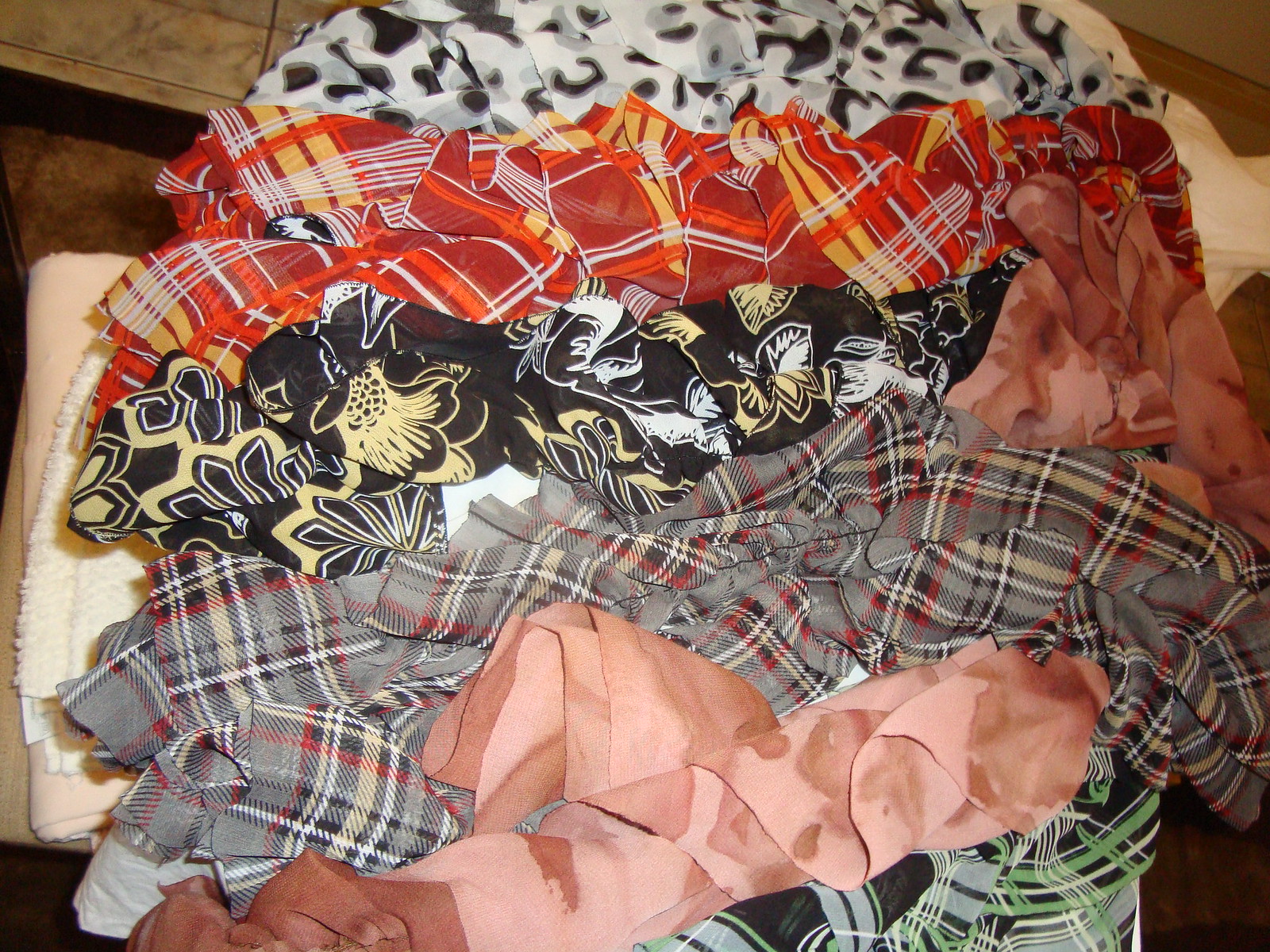The image depicts a collection of assorted fabrics tightly stacked in the foreground, resembling handkerchiefs or scarves, each with distinct patterns and textures. The setting appears to be within a house, which features a tiled floor with predominantly brown shades and a step or edge leading to an additional surface area, possibly carpeted. Toward the base of the fabric pile, there is a fuzzy, fur-like material layered with light pink fleece. Above these, the fabrics are meticulously arranged: 

1. A predominantly white fabric with black spots, reminiscent of a Rorschach test.
2. A red plaid fabric featuring intricate patterns of orange, yellow, and white lines.
3. A silky black fabric adorned with an ornate floral design in white and yellow, perhaps invoking an oriental aesthetic.
4. Another plaid fabric, primarily gray with hints of black, red, white, and tan, suggesting a robust wool or rougher cotton texture.
5. A pinkish-tan material with a somewhat camo-like appearance.
6. Additional fabric in the lower layers appears in green, gray, and black tones. 

All items in the image share a light, thin quality, possibly made from polyester silk or similar fabric, presenting a diverse and visually engaging textile array.